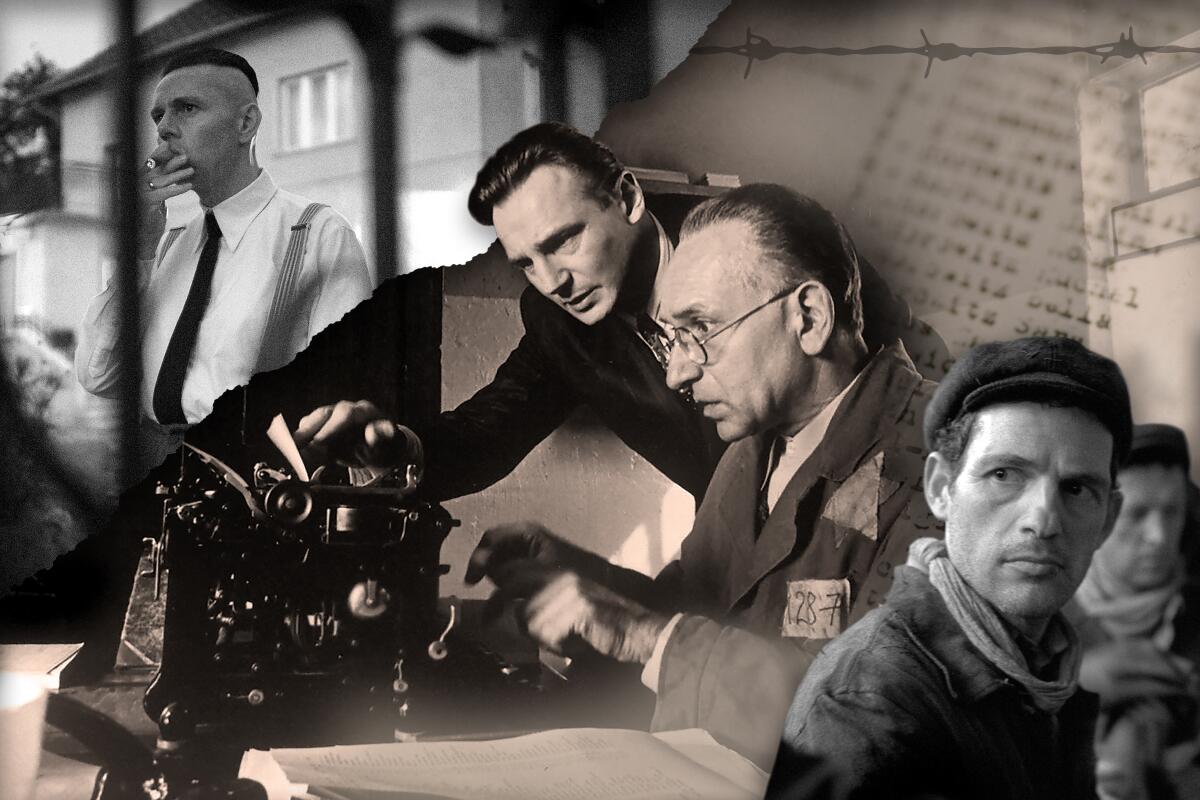The movie poster presents three diagonally-arranged, vintage-styled scenes: each image exuding a monochrome aesthetic with the central photo tinged in cream. The top left scene depicts a white male with short black hair, shaved sides, and wearing a white button-down shirt with a black necktie. He stands in front of a house, casually smoking a cigarette. The middle scene features an older man,, perhaps in his late 60s, wearing glasses and a button-down suit. He is seated at a black typewriter, focused on typing, while a slightly younger man in his late 40s, also in formal attire, leans over and points at the typewriter, assisting or collaborating in their task. This middle scene has a subtle sepia-toned hint, evoking a sense of historical importance. The bottom right scene captures a man with a black beret and a scarf around his neck, wearing a worn black jacket. Seated and gazing off to the side, he appears thoughtful, while other indistinct figures sit in the background, absorbed in their own subdued activities. Together, these scenes suggest a narrative set in a bygone era, potentially with historical or dramatic undertones.